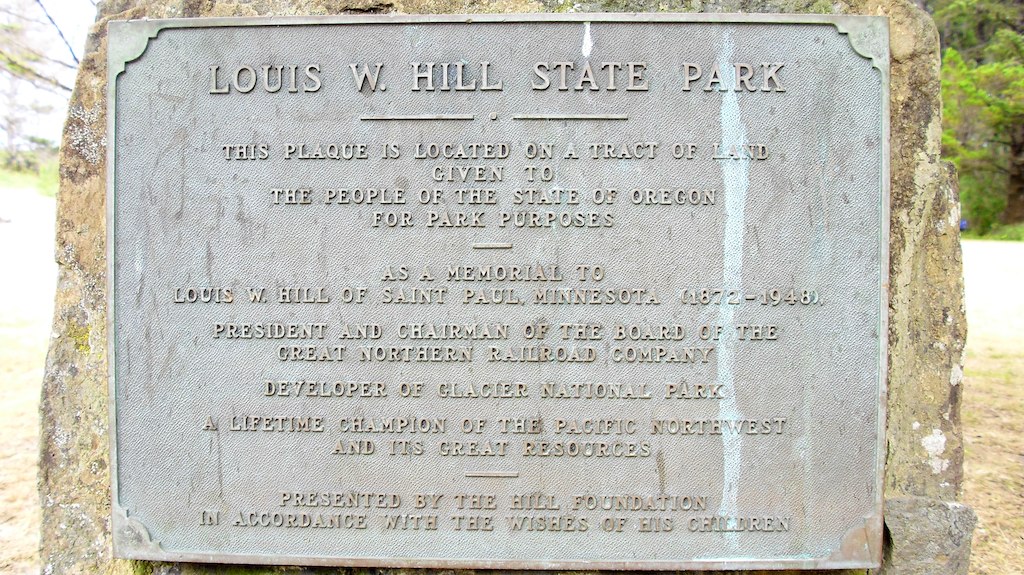This is a detailed photograph of a light gray stone or slate plaque engraved with writing, affixed to a large, multi-colored rock featuring shades of beige, gray, and brown. The plaque is framed with a narrow, engraved border. The text, centered both horizontally and vertically, reads:

**"LEWIS W. HILL STATE PARK"** 

Below this, a horizontal line divided by a dot separates it from the next section:

**"This plaque is dedicated and located on a tract of land given to the people of the state of Oregon for park purposes. As a memorial to Lewis W. Hill of St. Paul, Minnesota (1872-1948), president and chairman of the board of the Great Northern Railroad Company, developer of Glacier National Park, a lifetime champion of the Pacific Northwest and its great resources."**

An additional short horizontal line centers the final inscription:

**"Presented by the Hill Foundation in accordance with the wishes of his children."**

The plaque has visible imperfections, including various splotches and a prominent white streak running vertically down the right side. The background behind the rock hints at a green, cultivated park, enhancing the serene and respectful atmosphere of the setting.